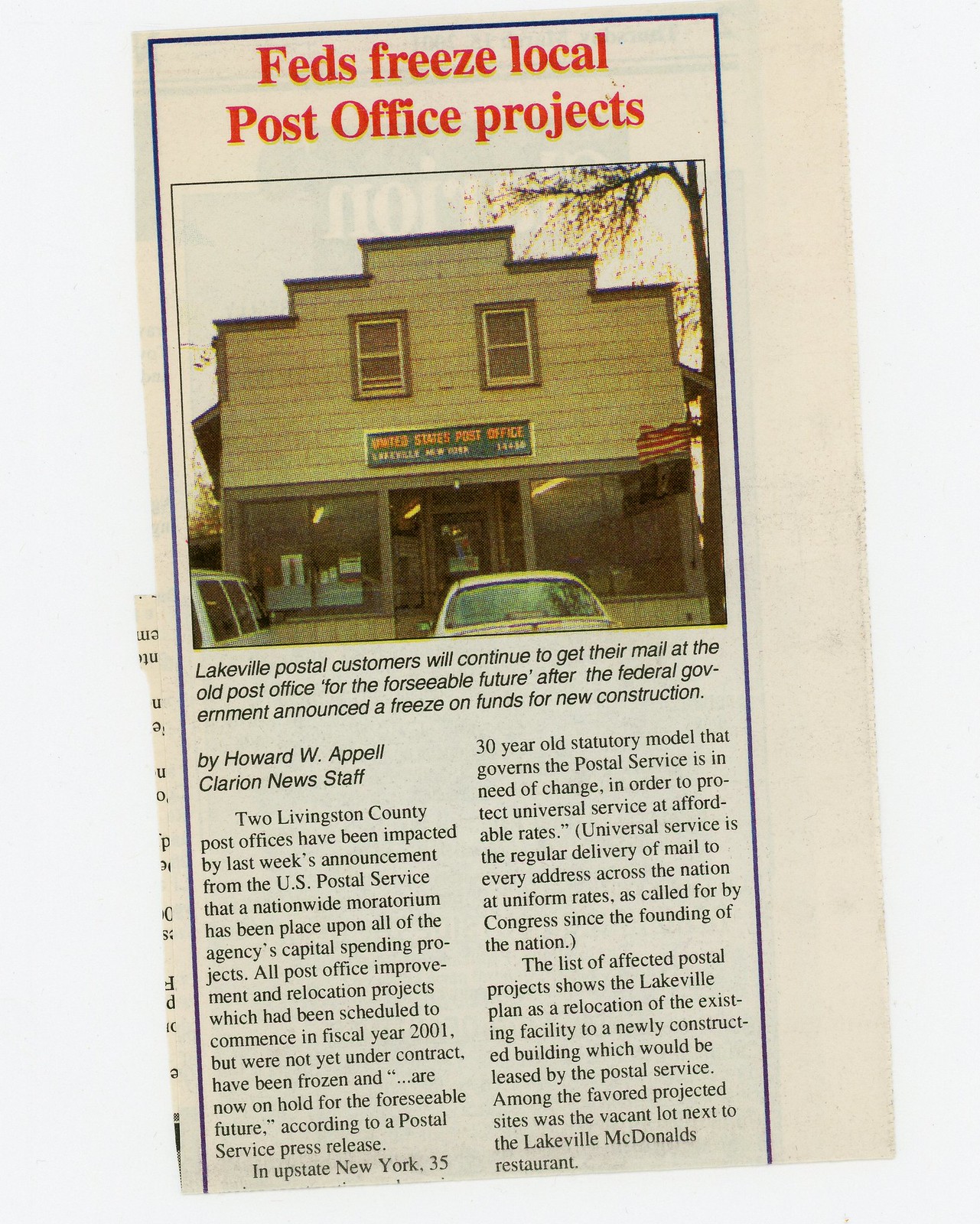This image is a snippet from an old newspaper article with a white backdrop. Dominating the top in bold red letters, it reads "Feds Freeze Local Post Office Projects." Below this heading is a color photograph showing the United States Post Office building, with visible signage indicating it is located in Lakeville, New York, and partially obscured text mentioning a zip code. In front of the post office building, a few cars are parked, and an American flag flutters.

The article's caption states, "Lakeville postal customers will continue to get their mail at the old post office for the foreseeable future, after the federal government announced a freeze on funds for new construction," authored by Howard W. Appel from Clarion News Staff. Detailing the content, it explains that two Livingston County post offices were affected by a recent nationwide moratorium announced by the U.S. Postal Service on all capital spending projects. This halt impacts all planned post office improvements and relocation projects scheduled to begin in fiscal year 2001 that were not yet under contract.

Additional details reveal that the 30-year-old statutory model governing the Postal Service is now seen as needing change to continue providing Universal Service at affordable rates. It further mentions that the Lakeville Post Office was planned to be relocated to a newly constructed building, potentially next to the local McDonald's, which would be leased by the Postal Service.